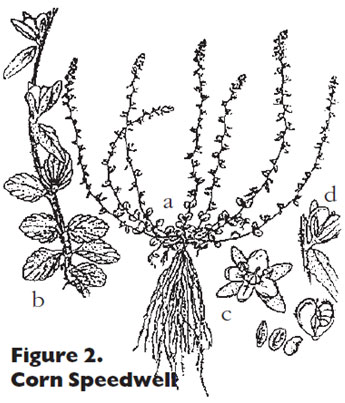This black-and-white drawing, titled "Figure 2.0, Corn Speedwell," depicts a detailed botanical illustration of the Corn Speedwell plant, rendered in black ink on a white background. The plant parts are labeled A through D, with each label corresponding to a distinct part of the plant. Label A shows the entire Corn Speedwell plant with multiple thin stems and sparse leaves, tapering to a bulkier root system at the bottom. B depicts a close-up of a stem with leaves branching off. C illustrates a small, delicate flower of the plant, while D represents the bulb or root section. Although the drawing style is somewhat crude, the diagram serves as an intricate and insightful botanical sketch, typical of illustrations found in a botanist's notebook.